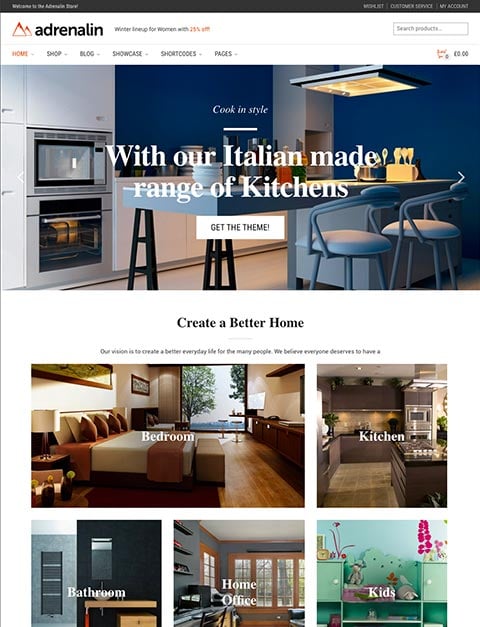**Detailed Caption:**

This image, sourced from the website Adrenaline (spelled A-D-R-E-N-A-L-I-N), features a variety of elements from their homepage. At the very top, there is a narrow black border, within which some text is present but illegible. In the top left corner of this black banner, there are some words, and in the right corner, there are three categories. While the first category is unclear, the second category reads "Customer Service," and the third reads "My Account."

Beneath this banner, two orange triangles resembling stylized mountains are positioned prominently. To the left of these triangles, the word "Adrenaline" is written in black font. On the right-hand side, there is a rectangular search box for looking up products.

Central to the image is a showcased photo of a kitchen. The kitchen features dark blue walls and white cabinets, prominently displaying an oven and what appears to be a microwave. The setting also includes an island with two bar stools. Overlaid on this photo is the text, "Cook in style with our Italian-made range of kitchens," written in an elegant font.

Below this text, there is a small white rectangle bearing the phrase "Get the theme" in black text. Directly underneath, the slogan "Create a better home" is displayed.

The lower portion of the image features five smaller photos arranged in a grid. The top row consists of two photos, and the bottom row contains three. Each photo is labeled in white text. The first photo in the top row is a bedroom labeled "Bedroom." The second in the top row is a kitchen labeled "Kitchen." The bottom row features a bathroom labeled "Bathroom," a home office labeled "Home Office," and a kids' room labeled "Kids."